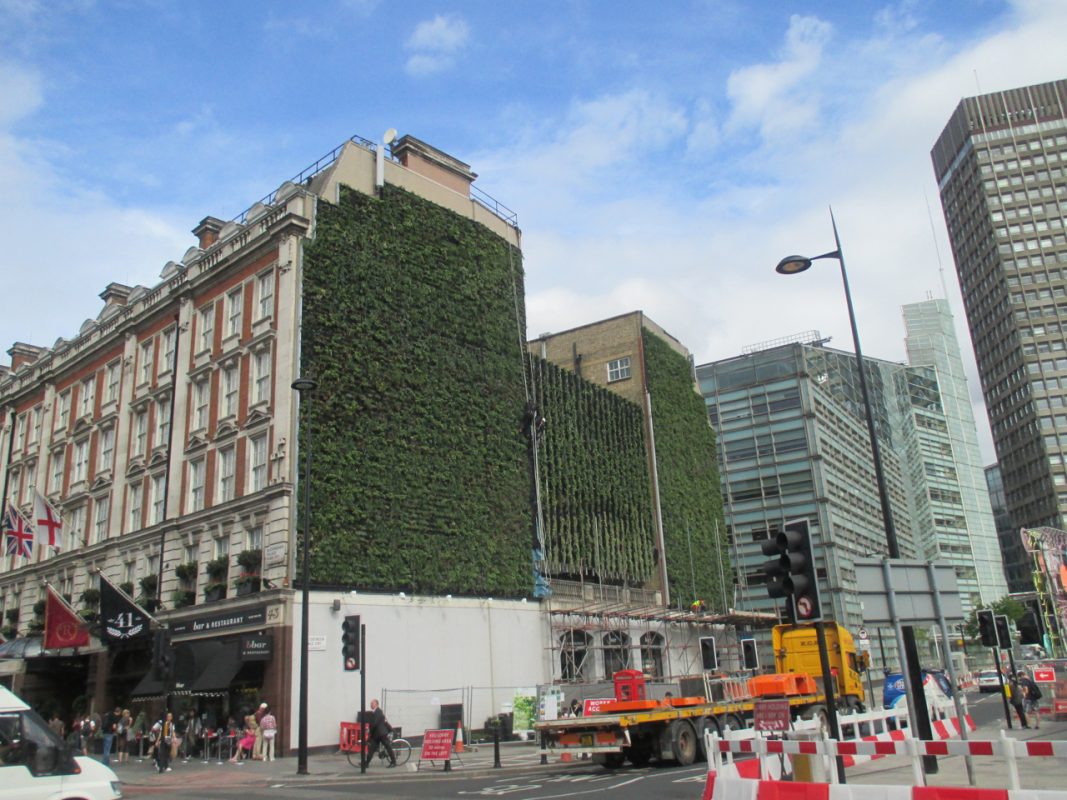This image captures a bustling street corner in a city block, likely in Britain. The focal point is an older building draped in lush green ivy on the corner, which houses a cafe with outdoor seating where patrons sit at tables under black umbrella canopies, sipping their drinks. The street is lively with pedestrians, including a man in a suit, walking along the sidewalk. On the left side, a bar and restaurant marked as number 41 displays British and possibly Scottish flags. The road adjacent to this building is closed off due to ongoing construction, evident by the red and white barricades and a prominent yellow construction truck at the blocked section. In the background, modern high-rise buildings with many windows contrast with the older architecture in the foreground. The sky is a bright blue with scattered white clouds, indicating a sunny day. Traffic signals and streetlights are visible, further adding to the urban atmosphere.